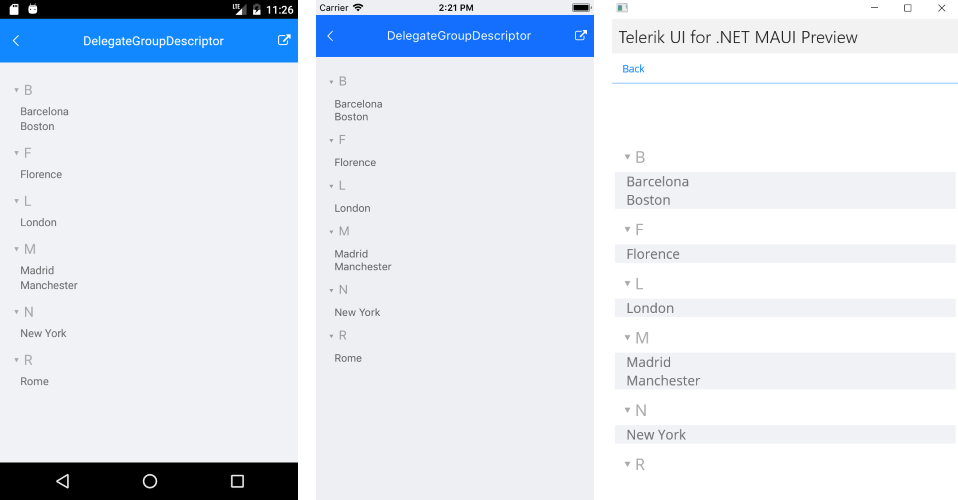The series of screenshots captures a mobile application interface, each displaying similar elements with slight variations. 

**Screenshot 1:**
- The top-left corner features a thin black bar with white icons, one resembling a computer chip and another looking like a cup of coffee, alongside battery strength and LTE indicators. The time displayed is 11:26.
- Below is a blue bar labeled "White Delegate Group Descriptor" with a back arrow and a box with an upward arrow.
- The main content area has a gray background with black text detailing different cities organized by letters:
  - B: Barcelona, Boston
  - F: Florence
  - L: London
  - M: Madrid, Manchester
  - N: New York
  - R: Rome
- At the bottom, there's a black bar housing white icons: a back triangle, a circle, and a square.

**Screenshot 2:**
- The top bar includes "Carrier" text, a black Wi-Fi symbol, the time 2:21, and a battery icon.
- A blue banner with white text reads "Delegate Group Descriptor" and includes a back arrow and a square with an upward arrow.
- The primary section mirrors the first screenshot, listing the same cities: Barcelona, Boston, Florence, London, Madrid, Manchester, New York, and Rome.

**Screenshot 3:**
- The top-left corner shows icons that look like a newspaper, a minus sign, a box, and an 'X'.
- The background is a white and gray pattern.
- The blue banner reads "Telerik UI for .NET MAUI Preview" and has an underline.
- The cities, now in gray boxes:
  - Barcelona
  - Boston
  - Florence
  - London
  - Madrid
  - Manchester
  - New York
  - The rest of the text is cut off, ending with the letter "R".

This detailed description offers a clear representation of the screenshots, emphasizing the consistent layout and slight differences in each image.